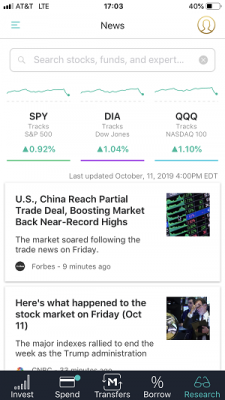Screenshot of an iPhone displaying a financial stock tracking app.

In the top navigation bar, the status information is shown:
- AT&T LTE signal with full bar strength on the left
- Current time displayed in the middle
- Battery indicator on the right showing 40% charge remaining

Below the status bar, the app interface begins, featuring:
- A header reading "News"
- A menu icon on the top left
- A user profile icon (depicted as a silhouette within a circle) on the top right

The main content includes:
- A search bar labeled "Search Stocks, Funds, and Experts"
- Three ellipses representing additional menu options

Below the search bar, a display of stock information:
1. SPY - Tracks the S&P 500
2. DIA - Tracks the Dow Jones
3. QQQ - Tracks the NASDAQ 100

Following the stock list, a series of news stories:
1. Headline: "U.S., China Reach Partial Trade Deal, Boosting Market Back Near Record Highs"
   - Summary: "Markets soared following the new trade news on Friday."
   - Source: Forbes, 9 minutes ago
2. Headline: "Here’s What Happened to the Stock Market on Friday, October 11th"
   - Summary: "The major indexes rallied to end the week as the Trump administration..."
   
At the bottom of the screen, a navigation menu includes buttons for:
- Invest
- Spend
- Transfers
- Borrow
- Research